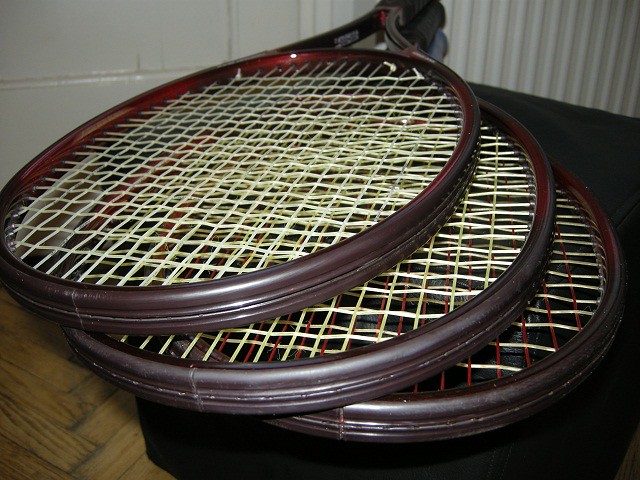The image is a close-up amateur photo of three stacked tennis rackets, likely taken indoors. The rackets lie on a black platform against a wooden floor composed of small sections of wood. All three rackets share an identical dark brown-burgundy frame. The string pattern on the rackets is a combination of white with alternating red vertical strings. The background includes a wall that appears to have a cinder block or tiled pattern. The photo's rectangular frame highlights the overlap of the rackets, emphasizing their lack of logos and the vintage aesthetic.